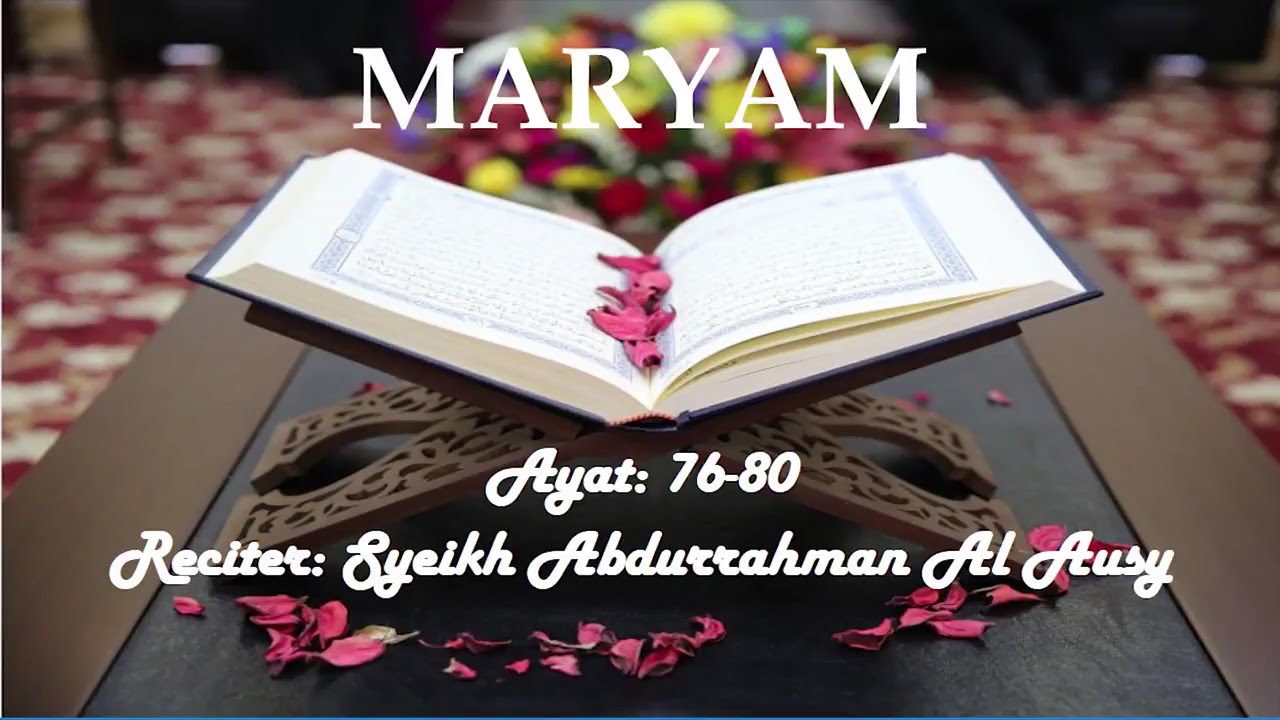The image displays an open book with a black cover resting at the center on a brown, heart-shaped stand adorned with cut-out patterns. The book's cream-colored pages are sprinkled with white flower petals along the middle crease. The stand sits on a black table with a contrasting white edge, and scattered red flower petals lie in front of the stand. Positioned atop a red carpet with white patterns. The top of the image features the word "Maryam" in large white letters, while beneath the book, "Ayat: 76-80" and "Reciter: Syeikh Abdurrahman Al-Ausy" are written in white text. The background is slightly blurred but reveals additional flowers and the patterned carpet.